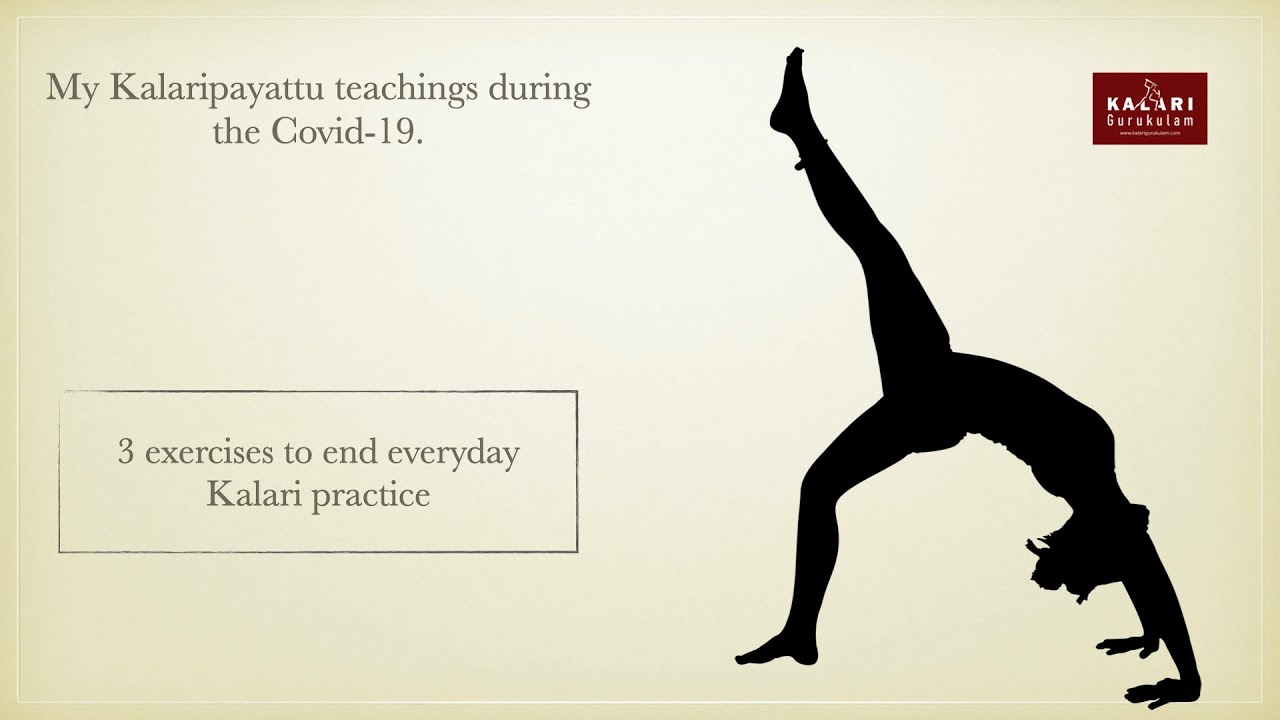This detailed drawing, likely an advertisement for Kalari practice, features a unique exercise against a pale peachy background. In the upper left-hand corner, the text "My Kalari Pilgrim Teachings during the COVID-19" is prominently displayed. A small maroon rectangle on the right side contains additional writing, possibly reading "Kalari Gurukulam." The lower left corner of the image includes a black-lined box with the words "Three exercises to end every day - Kalari practice." Dominating the scene, a solid black silhouette of a woman performing a backbend is centrally placed. Her palms rest on the floor behind her head, her right foot is firmly planted on the ground, and her left leg is extended upward in a graceful pose. Notably, there's a bracelet adorning her ankle, adding an elegant touch to her depiction. The exercise showcased exemplifies the limberness and strength developed through dedicated Kalari practice.